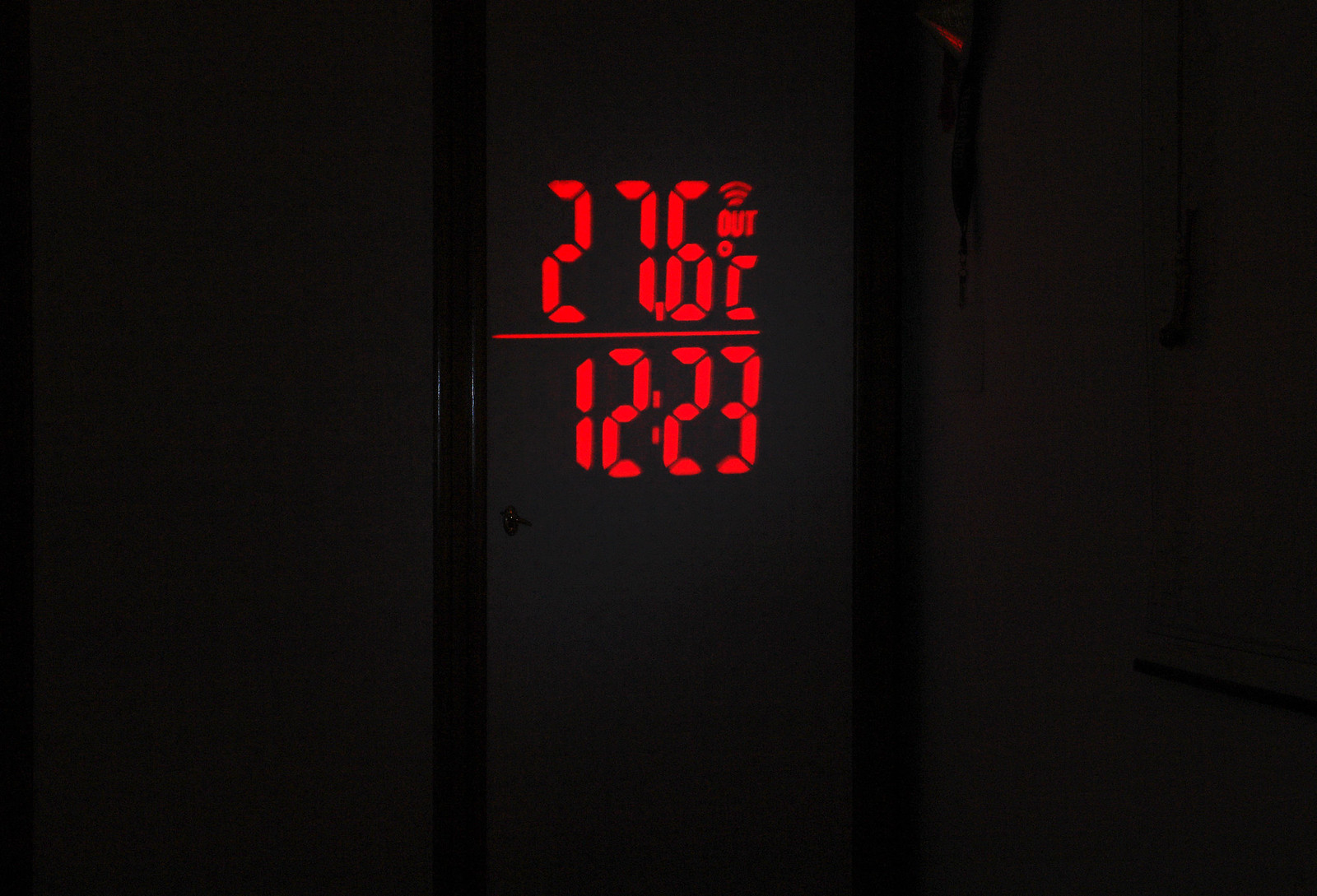The image depicts a dark, dimly lit room centered around a closed door. The door itself is a dark gray color framed by a shiny black door jamb. Dominating the scene is a bright red digital readout, akin to a digital clock, which stands out starkly against the black background. The display shows the temperature "27.6°C" with "out" written above it and a Wi-Fi symbol, reminiscent of connectivity bars, adjacent to it. A narrow red dashed line separates the temperature reading from the time below, which reads "12:23" in the same red text. Additionally, there is a subtle reflection in the upper right-hand corner, suggesting the presence of either two objects hanging on the wall or the edge of a window.